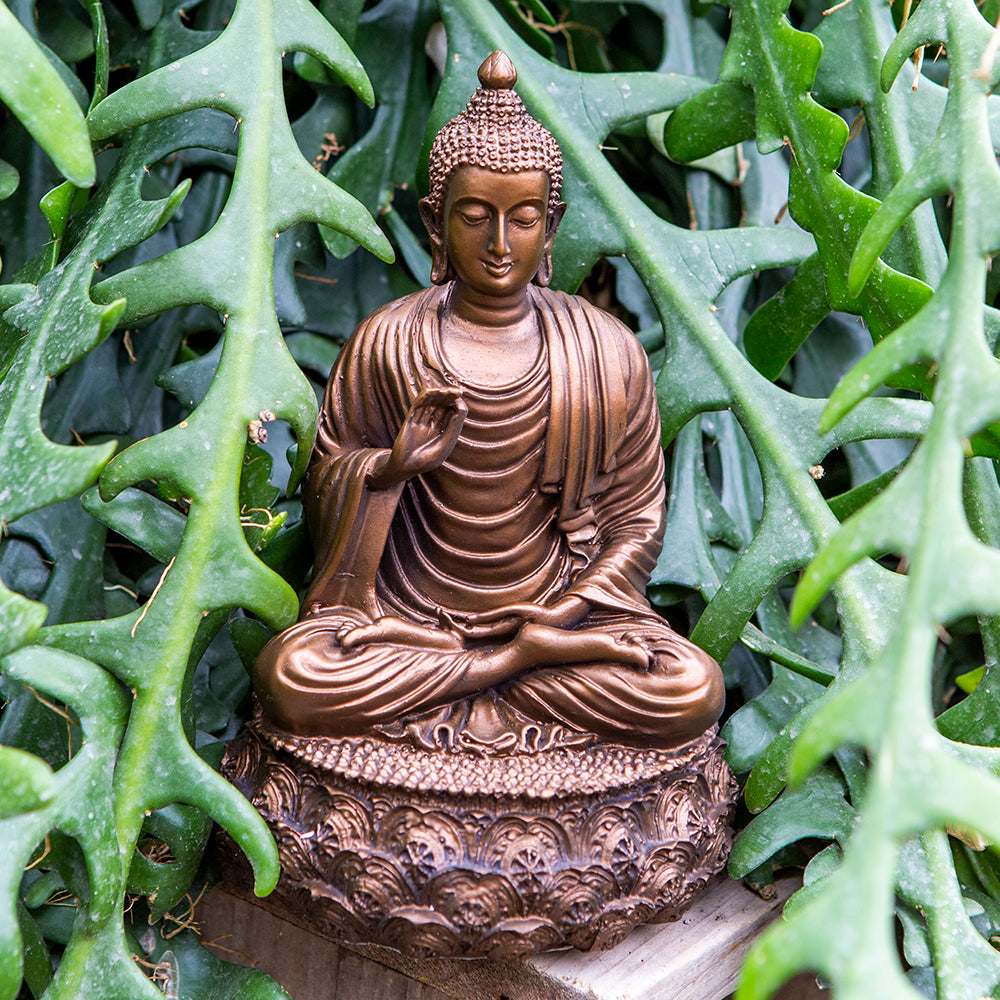This is a detailed, full-color photograph taken outdoors during the day, featuring a bronze Buddha statue as its central focus. The Buddha, depicted in a serene, meditative posture, is seated cross-legged on a small, bronze cushion. The left hand rests on his lap with the palm facing up, while the right hand is raised with the thumb and forefinger touching, forming the "okay" gesture. His hair is styled in a topknot, and his earlobes are elongated, adorned with hoop earrings. The statue, diminutive in size, rests on a wooden block surrounded by lush green foliage that engulfs the scene. The greenery is characterized by succulent leaves, which are thick, slightly wavy, and distinctly different from typical tree leaves. The background and foreground are both in sharp focus, capturing the intricate details of the statue and the vibrant beauty of the surrounding plants.